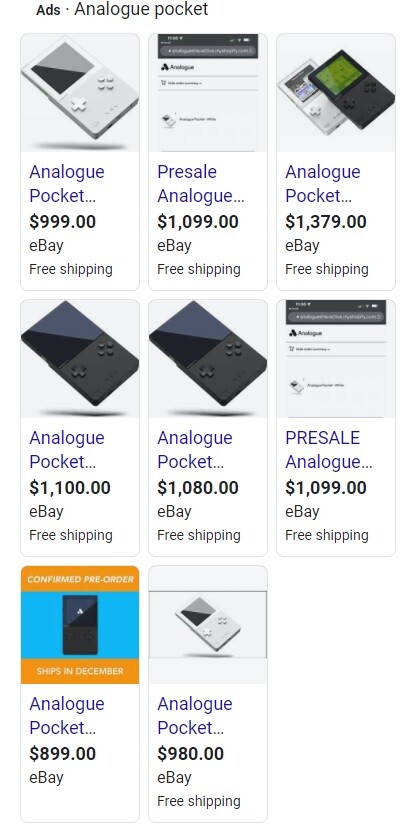The screen capture showcases a series of advertisements from an online site for Analog Pockets. At the top of the image, the words "ads • analog pocket" are written in black text. Below this heading, there are eight distinct images of Analog Pockets arranged in three rows: three images in the top row, three in the middle row, and two in the bottom row.

The first picture in the top row features an Analog Pocket with a silver frame, priced at $999 on eBay with the added benefit of free shipping. Directly beneath this, in the second row, the leftmost image displays a black Analog Pocket listed for $1,100 on eBay, which also includes free shipping.